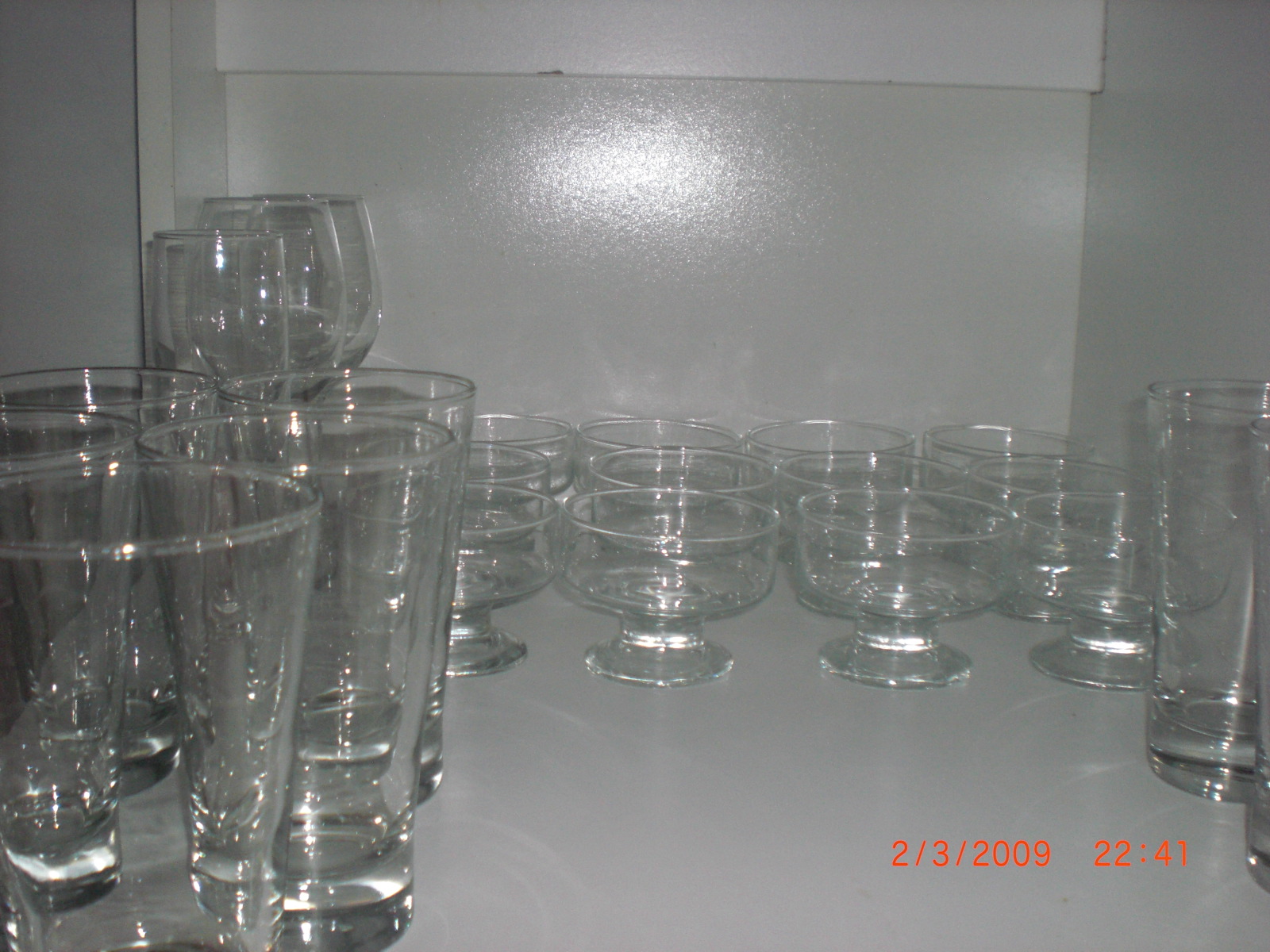The photograph captures the interior of a gleaming white display cabinet, brightly illuminated to showcase an assorted collection of glassware. The cabinet's glossy surfaces reflect a light source, enhancing the visibility of the objects within. To the left, tall highball and beer glasses are prominently positioned in front of a few roundly shaped wine and champagne glasses. Just to their right, several small, stemmed glass bowls that resemble snifters or dessert bowls for items like fruit cocktails are neatly arranged. Towards the bottom right of the image, there are a couple of shorter, regular drinking glasses, commonly used for iced tea or similar beverages. In the bottom right corner of the photograph, a red timestamp reads "2-3-2009 2241," marking the date and time the picture was taken.